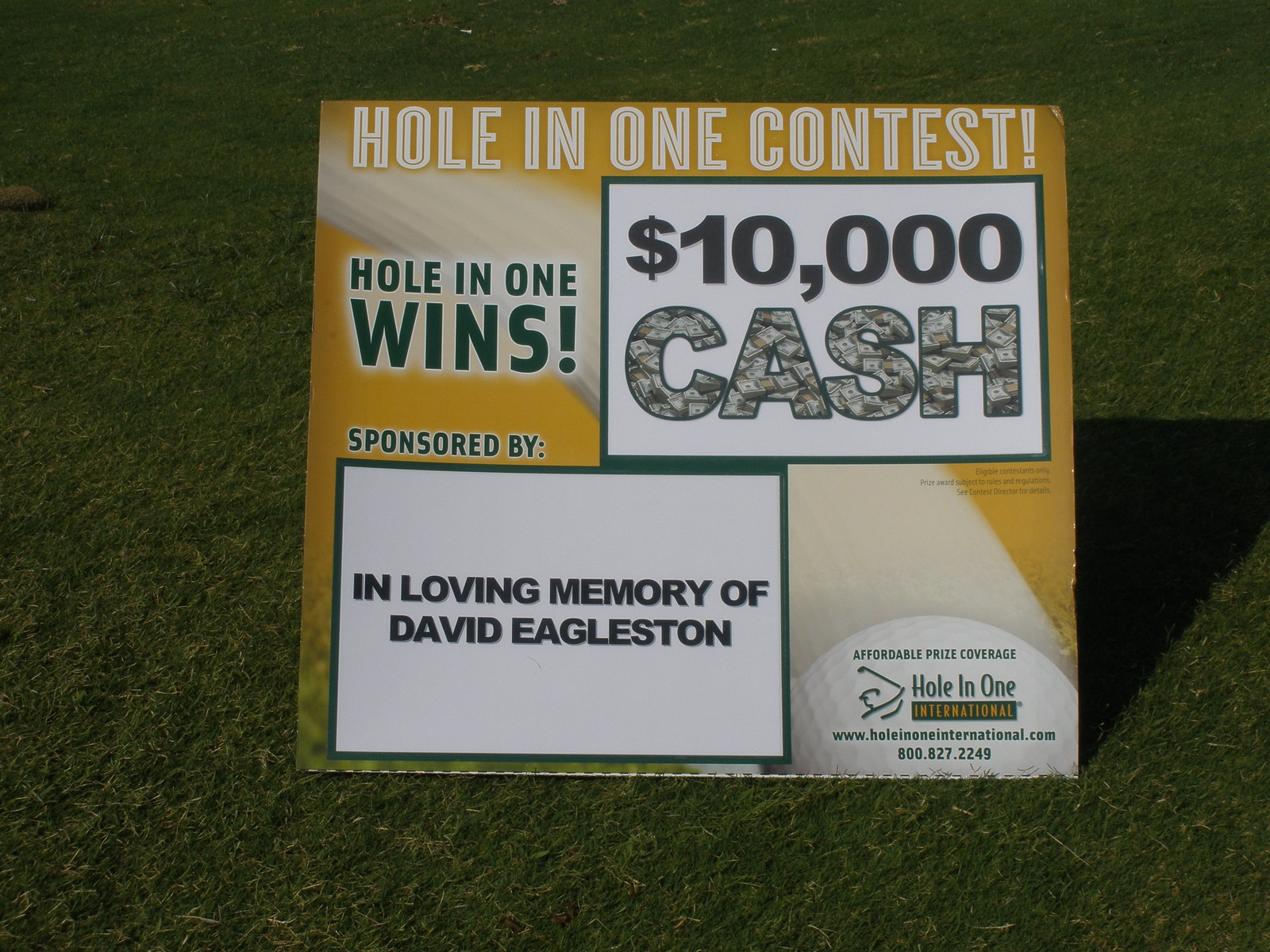This image features a postcard placed on the grass during an early part of the day, as indicated by the angle of the shadow behind it. The postcard announces a "Hole-in-One Contest" where a successful shot wins $10,000 in cash. The text on the yellow background highlights various denominations of money within the word "cash." This event is sponsored "In Loving Memory of David Eagleston," as noted prominently on the postcard. Additional information on the postcard includes sponsorship details from "Affordable Prize Coverage" and "Hole-in-One International." The website www.holeinoneinternational.com and the contact number 1-800-627-2249 are also provided. A golf ball is noticeably positioned behind the postcard, adding to the thematic elements of the golf tournament. The simple, yet poignant image underscores the memorial nature of the contest.